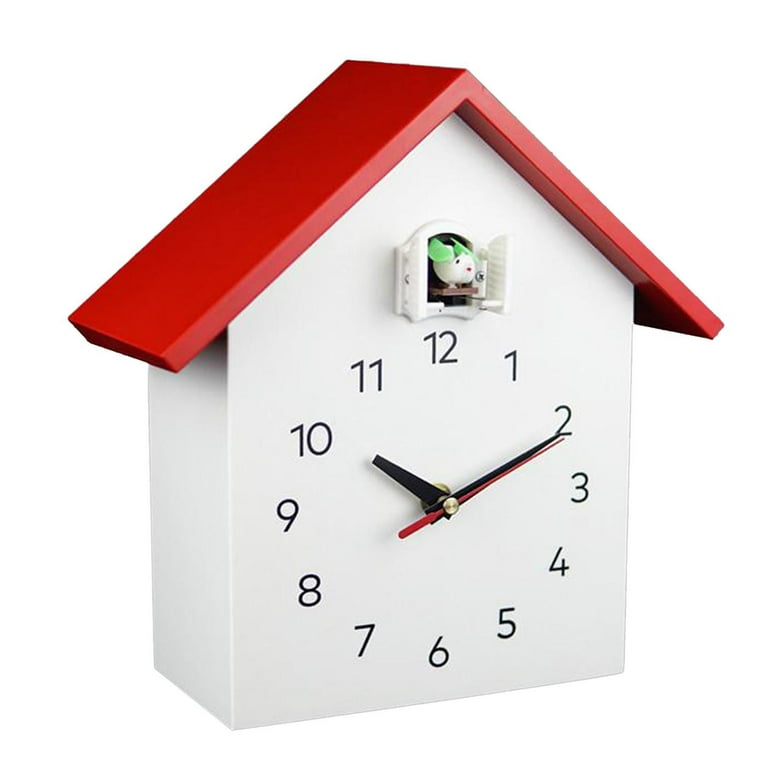The image features a unique cuckoo clock designed in the shape of a house, emphasizing its simple and smooth plastic construction. The clock has a vibrant red, sloped roof and a white body, creating a clean, minimalistic look. The face of the clock displays numbers 1 through 12 in a sans serif style, arranged in a circular pattern typical of analog clocks. 

Three hands are present: the hour and minute hands in black, and a red second hand. They all stem from a central gold-colored rivet. The hands are positioned to show the time as 10:10. Above the clock face, a small plastic window with white doors is open, revealing a unique 'cuckoo' mechanism—a small white mouse with black eyes, green markings, and large green ears, appearing instead of a traditional bird. This clock, likely featured in an advertisement, shows the mouse striking, adding an element of curiosity and charm to the timepiece.